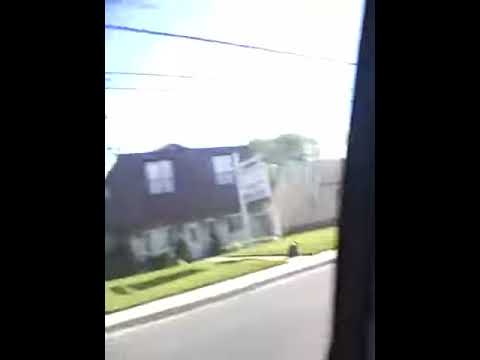This photograph, likely taken from inside a moving vehicle or through a window framed by black curtains, depicts a somewhat run-down, two-story white house with a red roof and large windows. The house is situated across a paved gray street, bordered by a neatly manicured green lawn and a white sidewalk. In front of the house, there is an indistinct sign that may suggest it's for sale or could be related to a business. 

The shot features a wide black margin on both the left and right sides, possibly indicating it was taken through a pane with a vertical support or window frame in view. There are no people or animals present, and the image quality is poor and slightly blurred, possibly from motion. Above, three telephone wires cut across a bright sky, which radiates a white flash possibly from sunlight or a camera's effect, hinting at a bright, sunny day. In the background, a small section of blue sky peeks through. Another white house can be seen to the right, adding to the suburban setting.